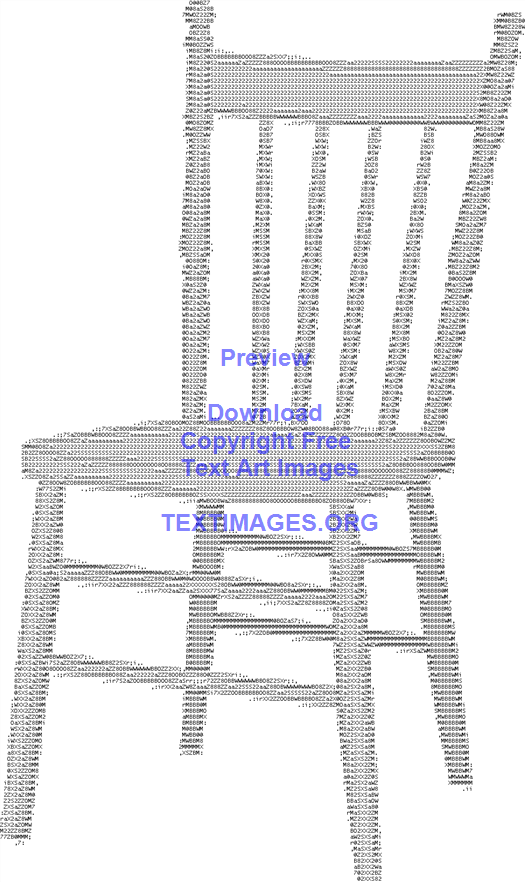The image is a detailed digital illustration of a wooden chair, created using a combination of binary code, letters, and numbers. The chair, reminiscent of an old-fashioned, uncomfortable wooden seat often found in elderly homes or outdated decor, features a backrest made of four dowels and has two horizontal supports between both the front and back legs. It is meticulously arranged so the darker characters depict the back legs, providing shading and a sense of depth. The chair's intricate design includes a carved top with knob-like details and showcases rails with gaps between them for the upper and lower back support. The entire composition rests against a white background, with the black and gray tones of the text art forming the chair's silhouette. Overlaid at the center of the image in blue font are the words "Preview, Download, copyright-free text art images" and below it, the source "textimages.org."